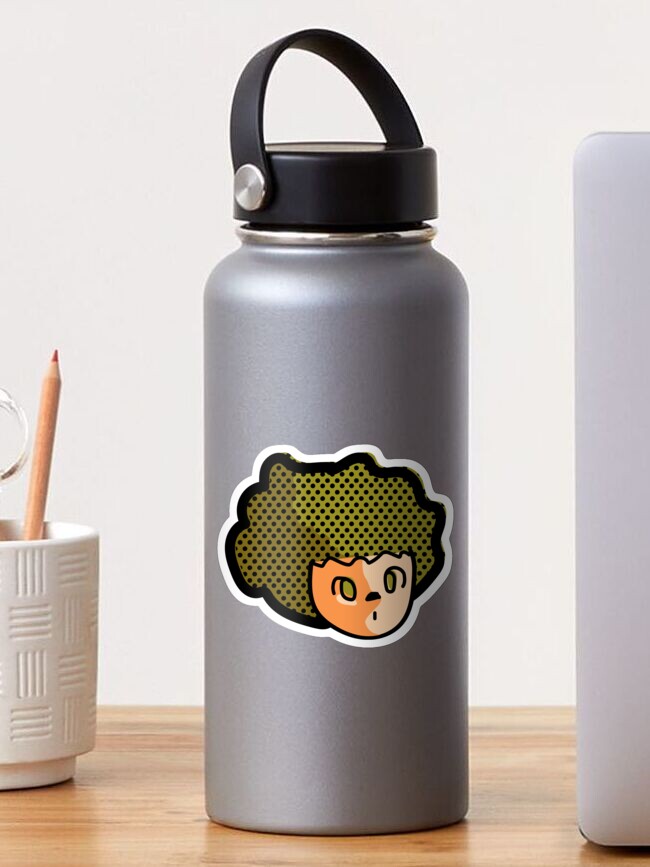This is a detailed, marketing-style photograph of a slender, cylindrical silver stainless steel thermos, centrally positioned on a light, wooden surface with a plain white wall in the background. The thermos has a black screw-on cap equipped with a hinged handle running horizontally across the top. Adorning the middle of the thermos is a sticker featuring a cartoon character. The character is a little girl with a button nose, wide eyes, and a small mouth, her hair depicted in a green and black polka-dotted afro with white and black outlines.

On the left side of the photograph, partially cut off by the edge, is a white ceramic pencil cup holding an upward-pointing pencil and the tips of a pair of scissors. To the right is a partially visible silver object resembling a laptop lid, likely a MacBook, which is the same height as the thermos but cut off by the photo's edge.

Overall, the photograph is vertical, making it significantly taller than it is wide. The clean composition highlights the main subject — the thermos with its distinctive cartoon sticker — while giving a glimpse into the surrounding objects, suggesting a casual workspace setting.